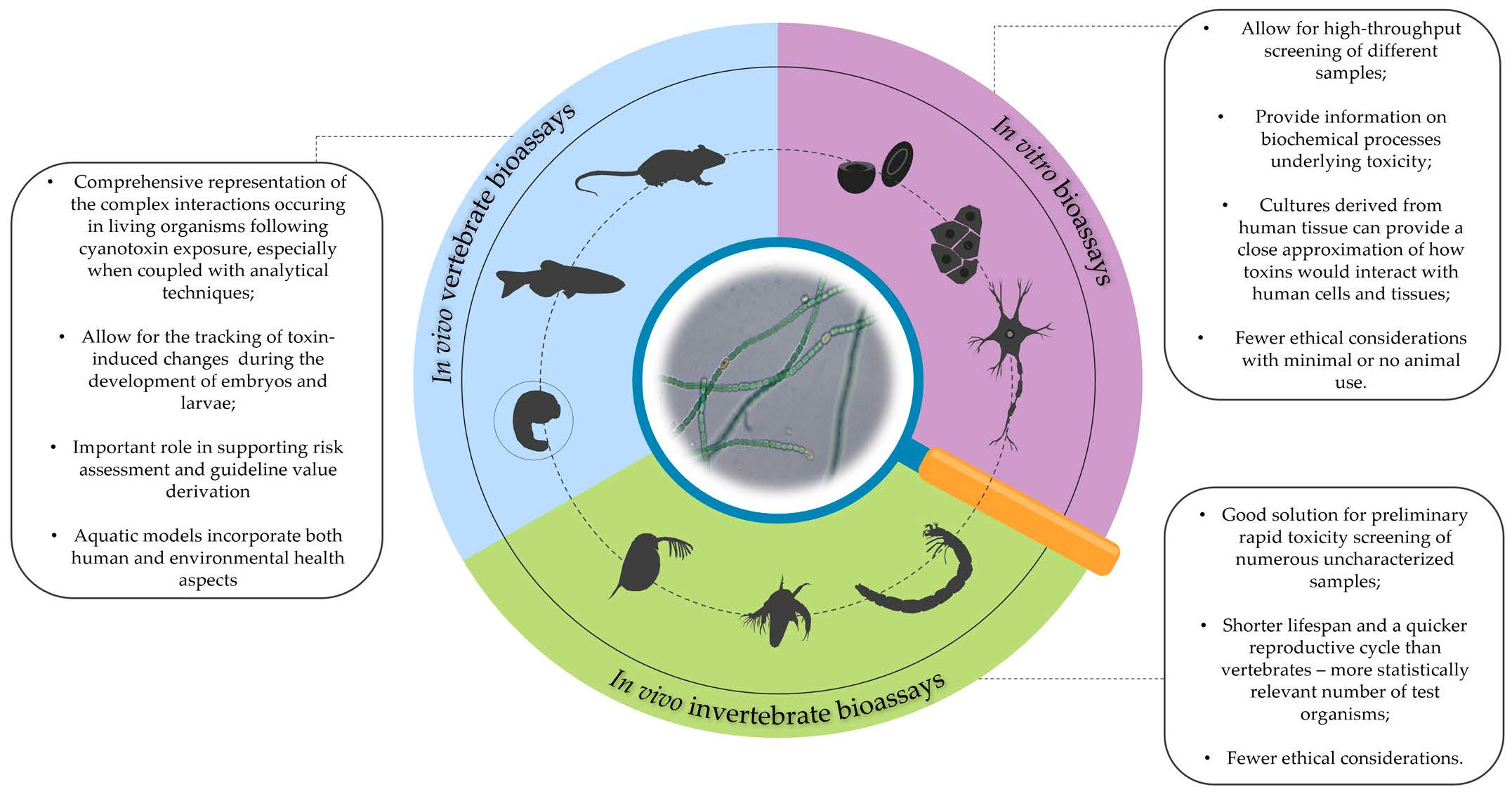This textbook diagram illustrates various bioassay methods categorized into three colored sections within a circle, each with detailed descriptions and illustrations. The blue section, labeled "In Vivo Vertebrate Bioassays," contains representations of a mouse, a shark, and a curved organism, highlighting complex interactions in living vertebrates exposed to cyanotoxins, essential for comprehensive risk assessment in human and environmental health. The purple section, labeled "In Vitro Bioassays," showcases images of cells, including a neuron, a red blood cell, and a skin cell, emphasizing high-throughput screening and biochemical process analysis with minimal ethical concerns. The green section, labeled "In Vivo Invertebrate Bioassays," features illustrations of a worm and other invertebrates, noting the advantages for rapid preliminary toxicity screening due to their shorter lifespans, quicker reproductive cycles, and lower ethical considerations. Each section includes a block of text with arrows pointing to the respective colored area, providing detailed explanations of the depicted assay methods. At the center of the diagram is a magnifying glass, symbolizing the focus on microbiological examination.